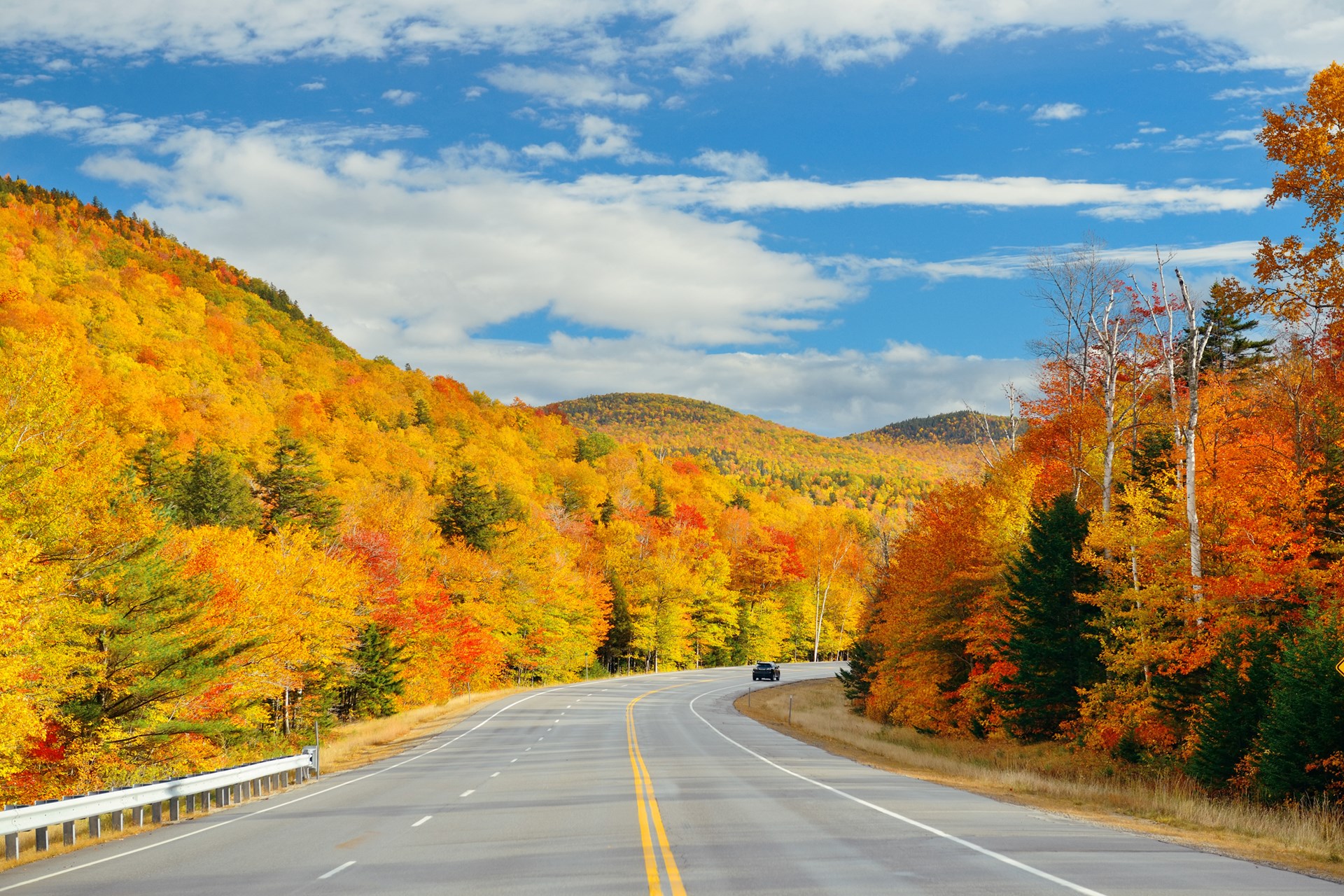This photo captures a vivid autumn scene, showcasing a three-lane highway that winds through a picturesque mountainous landscape. The season is fall, evident from the kaleidoscope of colors adorning the trees—vibrant oranges, yellows, reds, and lingering summer greens. The trees are in the midst of shedding their leaves, signaling the transition between fall and winter. The bright, clear day is adorned with several white clouds against a striking blue sky, enhancing the overall beauty of the scene without detracting from the intense fall colors. The road, marked by double solid lines in the center, appears mostly empty save for a single small black car heading away from the viewer. A guardrail lines the left side of the highway, which carves through the forested hills. The temperature seems comfortably crisp, around 50 degrees Fahrenheit, adding to the refreshing ambiance. This serene moment is a perfect capture of the breathtaking splendor of an autumn day.